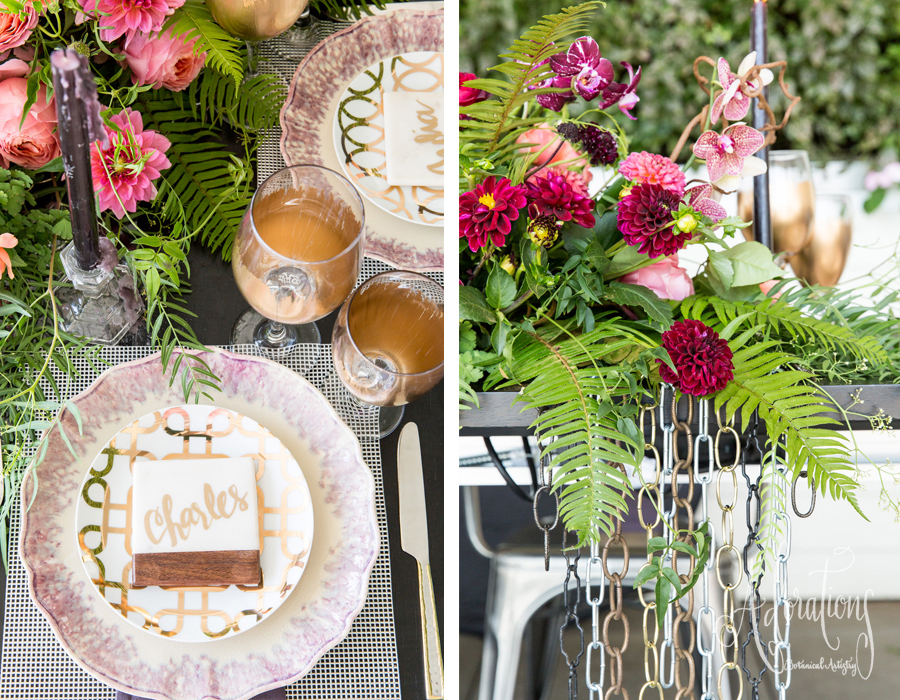The image, likely an advertisement for a wedding planner or a high-end event setup, features two side-by-side vertical photographs separated by a white rectangular border. On the left, a top-down view displays an elegant place setting with two decorative plates: one with a lilac design on a scalloped edge and the other with a gold pattern on the white center, trimmed in pink that matches the flowers on the table. A gold-engraved napkin bearing the name "Charles" rests elegantly atop one plate, while another napkin, partly cropped and unreadable, possibly displays a second name, perhaps "Andrea." Positioned between the plates are two goblets filled with a clear gold liquid, likely wine or brandy, and accented by a glass candlestick holding a black candle. Pink chrysanthemums and green fern leaves intricately decorate the table, adding a fresh, floral touch. The right photograph complements the left, displaying a sophisticated floral arrangement with cascading bronze, silver, and gold chains. The arrangement includes green leaves and flowers in shades of dark magenta and pink, some with hints of white. A signature in cursive, though unreadable, adorns the lower right, signifying a photographer's credit or branding. The blurred background suggests a garden setting, enhancing the romantic and luxurious ambiance.